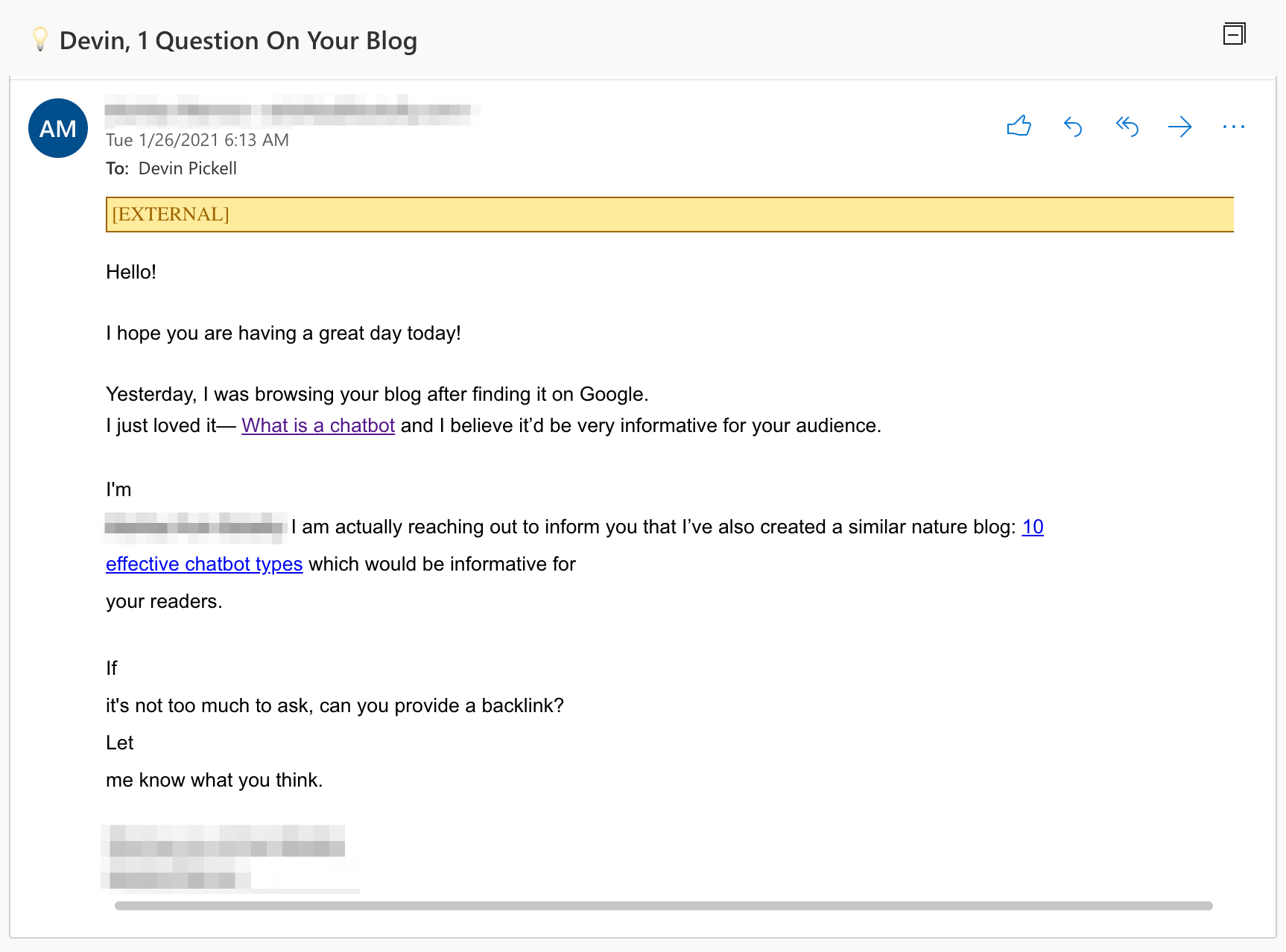The image depicts an email screenshot. In the upper-left corner, there's a lightbulb icon alongside the text "Devon." Below this, the subject line reads "One question on your blog." Adjacent to this, there's a blue circle with "AM" inside it, and next to it, partially blurred, appears to be the sender's email and name. The email was sent on Tuesday, January 26, 2021, at 6:13 AM, addressed to Devon Pickle.

The email starts with a friendly greeting: "Hello, I hope you're having a great day." The sender explains they discovered Devon's blog via Google and enjoyed it. The primary inquiry of the email is underlined and in a different color, asking, "What is a chatbox?" The sender believes discussing chatboxes would be informative for Devon's audience.

The sender, whose name is also blurred, mentions that they have created a similar nature blog. This section highlights their work titled "10 Effective Chatbox Types," which is underlined and colored in blue. The sender then requests a backlink to this blog post, concluding with "Let me know what you think" before their name is blurred again at the bottom.

A light green line is present at the very bottom of the email.